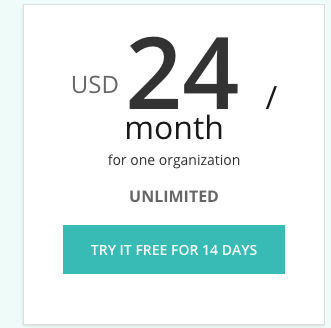The image showcases a pricing plan for a service. At the top of a white square, the text "USD" is displayed in gray letters. To the right of "USD" are the numbers "24" in a large, bold black font, followed by a small black slash. Directly below "24," the word "month" is written in standard, lowercase gray text, indicating the cost is "$24 per month." Underneath this, the additional description "for one organization" appears in gray text. Below this phrase is the word "UNLIMITED" written in all uppercase letters. At the bottom of the square is an aqua green rectangular button with white uppercase text that reads "TRY IT FREE FOR 14 DAYS."